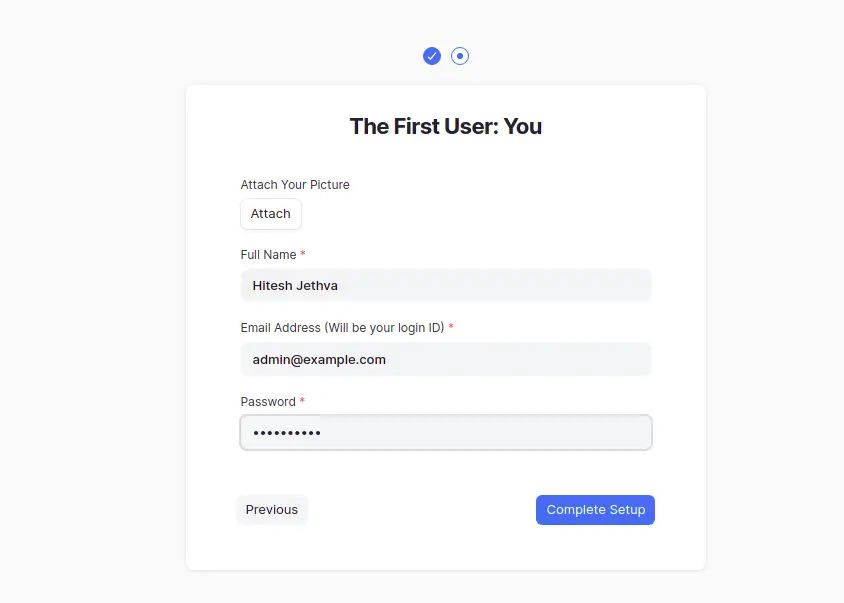A detailed and cleaned-up caption for the described image:

The screenshot captures a straightforward login setup screen with several key elements. At the top of the screen are two circles: the first contains a checkmark, and the second features a small square. Below these indicators, centered on the screen in black text, is the label "First User: You."

The next section invites the user to "attach your picture," accompanied by a button labeled "Attach." Proceeding downward, the form requires a "Full Name," as indicated by a red asterisk marking it as a mandatory field. In this field, the name "Hitesh Jethva" is entered.

Further down, another mandatory field is labeled "Email address will be your login ID," marked with a red asterisk. The placeholder text within this field shows "admin@example.com." The final required field is for the "Password," again denoted by a red asterisk. The password entered here is masked by a series of asterisks for security.

At the bottom of the screen are two buttons: "Previous" on the lower left, and a blue "Complete Setup" button with white text on the lower right. The overall design is clean and functional, ensuring users can easily navigate through the initial login setup process.